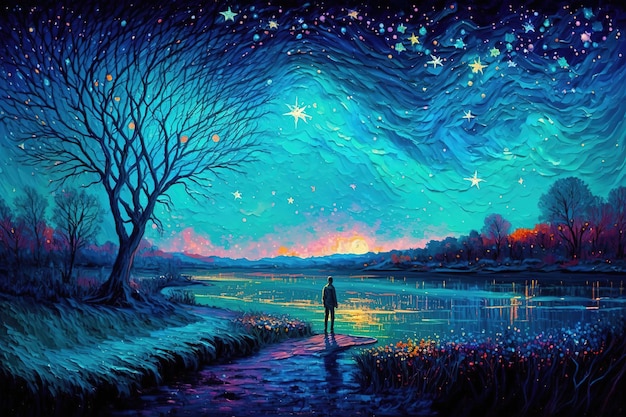This painting features a lone figure standing on the bank of a tranquil water body, which appears to be either a pond or a river opening into a larger lake. The central figure, silhouetted and facing away from the viewer, gazes out over the water, immersing themselves in the stunning nighttime scenery. The sky, a rich tapestry of colors, begins with a deep black at the top, dotted with sparkling stars, and fades through dark blue and teal to a lighter blue hue. Just above the horizon, hints of orange and red suggest the impending sunrise or a distant glow. On the left of the scene, a large, leafless tree stretches its bare branches upwards, partially blending with wavy, horizontal cloud lines adorned with a plethora of brightly colored stars. This tree stands on a grassy embankment, juxtaposed against a backdrop of more densely packed trees that hint at a forest beyond. To the right of the figure, a field of flowers adds to the lush, surreal quality of the scene. The water in front of the person reflects the myriad colors of the sky, with light blue tinged with yellow reflections. Overall, the blend of vivid hues and dreamlike elements evoke a whimsical, almost otherworldly feel to the artwork, reminiscent of a starry night.